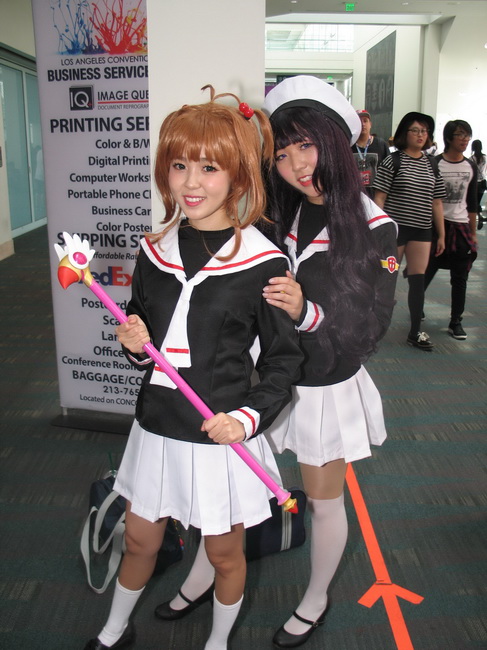In the image, two Asian girls are dressed in matching outfits, reminiscent of characters from Sailor Moon. One girl, with brown hair, stands slightly in front holding a long pink stick topped with a plastic chicken head. The other girl, with black hair, stands behind her at an angle and gently places her hands on the brown-haired girl's shoulders. Both of them are wearing dark shirts with white ties accented with red, sailor-style tops, white short pleated skirts, long white socks, and black Mary Jane shoes. The girl standing behind also dons a white sailor hat. They appear to be at a comic-con event, as suggested by the background scene featuring a banner promoting business services with a printer, and other attendees walking forward on the right side of the frame. The setting is lively, with an orange arrow line on the ground and people in the distance.